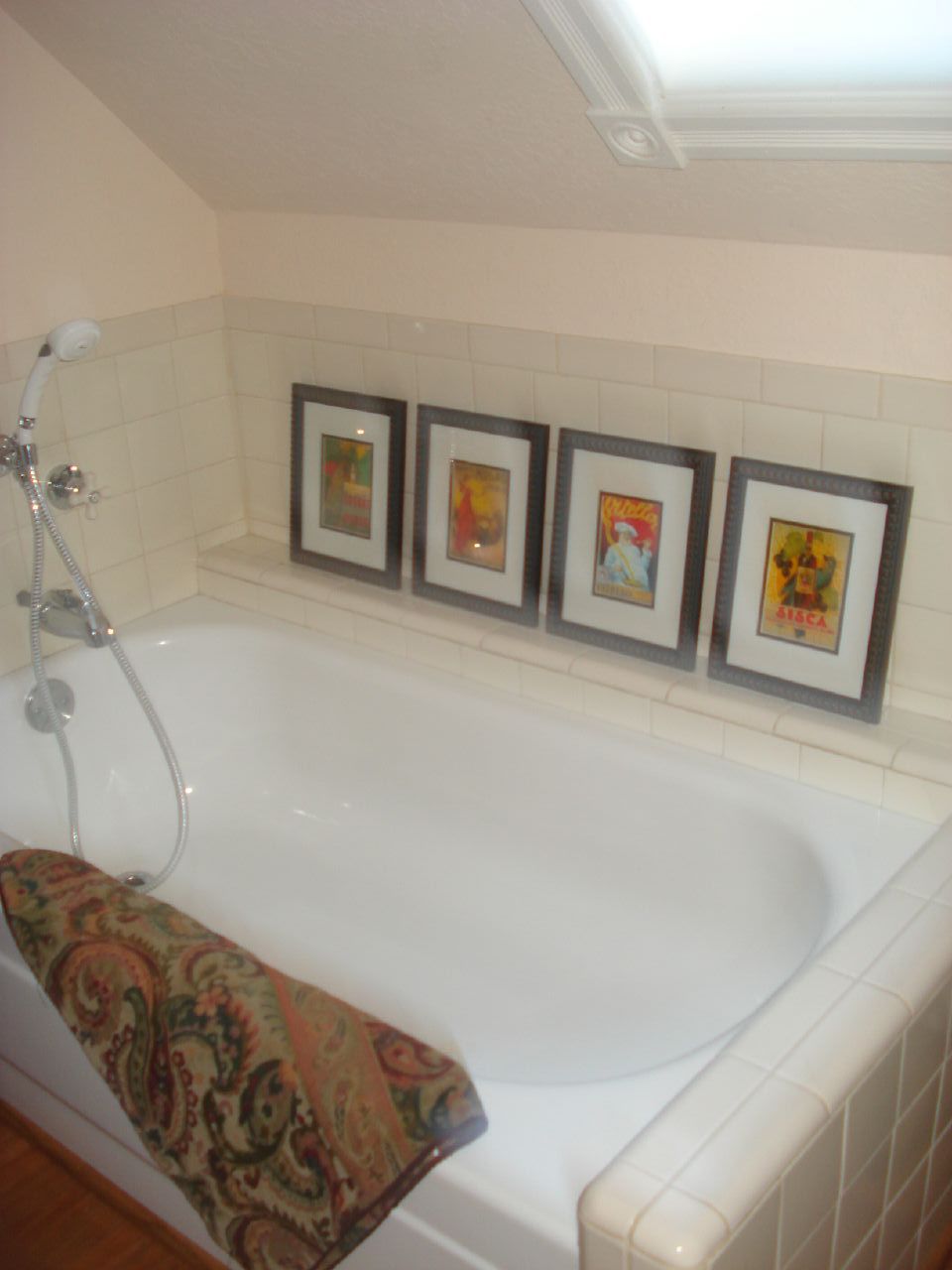This detailed photograph captures a spacious, pearly white, ceramic bathtub situated diagonally from the bottom right corner towards the middle left of the frame. The tub features an oval-shaped deep opening and is framed by white tiles. At the far end on the left, a short concrete barrier, painted white, rises just above the tub. The bathroom has no enclosing shower doors or walls.

A silver faucet with matching handles for water control is installed at the left end of the tub. There's also a handheld shower head with a long, flexible cord. The shower head is white at the part where the water exits. Adjacent to the faucet, a green wall, extending from an inch at the left, serves as the backdrop. This wall hosts four small photographs framed in black, each with indistinct artwork, bordered by white.

The bathtub's edge features a texture-rich bath mat draped over it, resembling an oriental rug in hues of tan, green, and an orange-reddish color. Additionally, a small, reddish-brown rug is visible on the floor in the bottom left corner of the image. The ceiling above showcases a white-trimmed skylight positioned towards the top right section of the frame, bathing the bathroom in natural light.